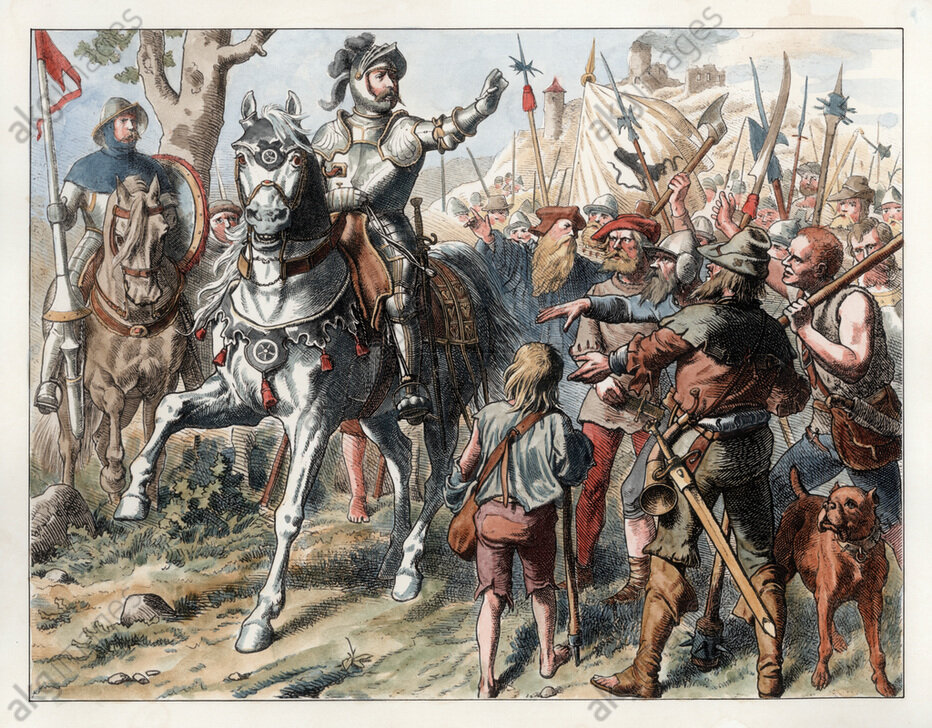The image is an antique illustration of a medieval campaign featuring a central figure, a knight in shining armor seated atop a large white horse adorned with silver embellishments. The knight, in full body armor, is raising his left arm in a halting gesture towards a crowd of peasants. These peasants, appearing disheveled and weapon-wielding with axes, spikes, and sticks, surround the knight in what seems to be an atmosphere of unrest or protest. Notably, a few of the peasants are barefoot, underscoring their poverty. Among the crowd, a peasant child with longish hair, short pants, a shirt, and a bag slung over his shoulder stands to the right of the knight, while a small dog is visible in the lower right corner. To the left of the white horse, another knight on a brownish horse holds a lance adorned with a small red and white flag. This second knight wears a partial helmet that does not cover his face entirely, and a tree is visible behind him in the scene. Additionally, a castle looms in the far distance atop a hill, completing the backdrop of this vividly detailed medieval confrontation.